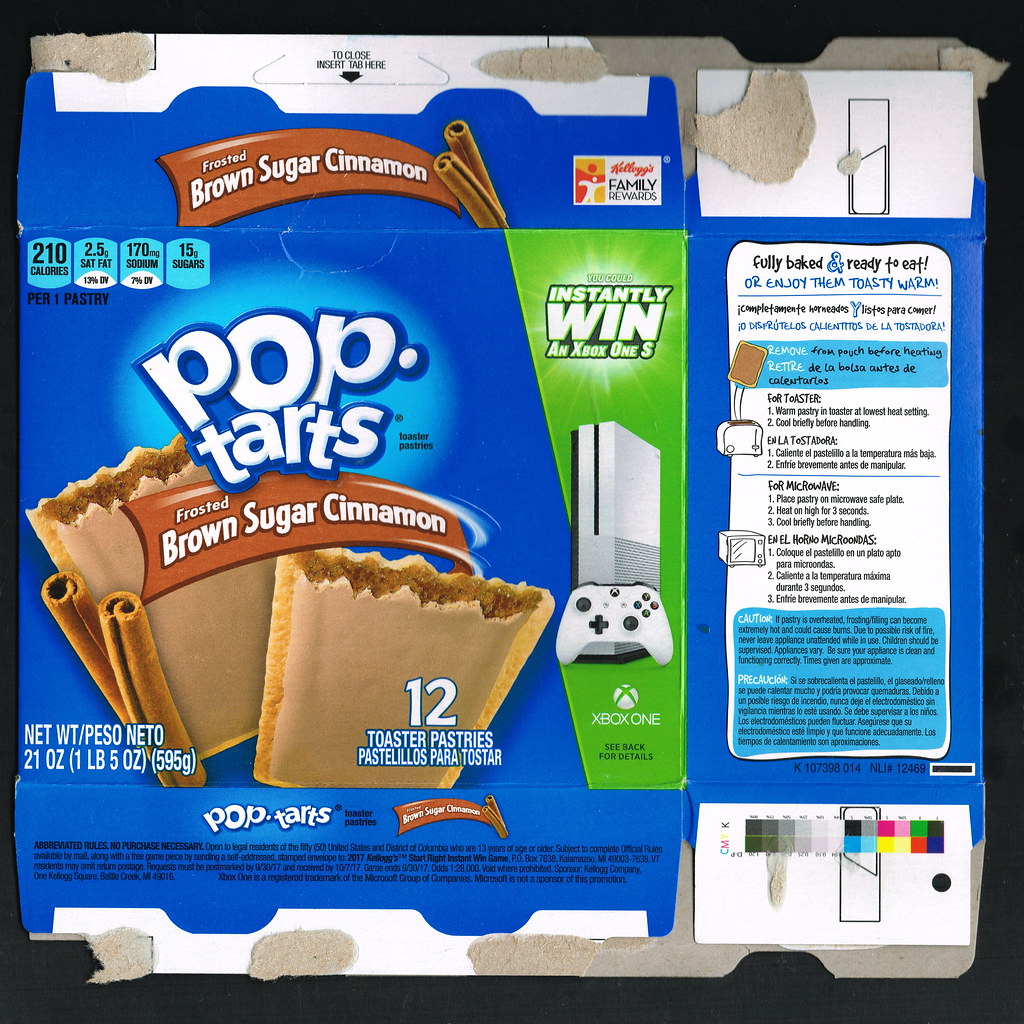In this image, set against a black background, there is a blue Pop-Tart box that has been opened and flattened to reveal both the front and side panels. The front of the box prominently displays the Pop-Tarts branding in large white letters. Below the brand name, there is a brown rectangle with white letters indicating the flavor: "Brown Sugar Cinnamon," accompanied by an illustration of two cinnamon sticks. Toward the side of the box, a green rectangle with white text announces an "Instant Win an Xbox Series X" promotion, featuring an image of the Xbox. The box graphic also shows an illustration of two brown sugar cinnamon Pop-Tarts and includes detailed instructions on how to prepare them, depicted neatly on the side panel.